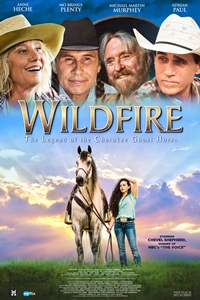The movie poster for "Wildfire: The Legend of the Cherokee Ghost Horse" features a dramatic sky background with gradients ranging from blue to purple, transitioning into a sunset behind the main figures. Central to the poster is a young woman with brown hair, dressed in a green t-shirt and jeans, standing next to a white horse with a black mane and a brown saddle. She holds the reins of the horse, which is positioned on the left, while she stands to the right.

Above the title "Wildfire," displayed in a goldish tint, are the faces of the four main actors: an older woman with a tan hat (possibly Ann Heche), a man with a black hat, another man with a beard and gray hair wearing a black cowboy hat, and a younger man with a white cowboy hat. Although the actors' names such as Mitchell Martin Murphy and Adrian Paul are not clearly legible, the composition emphasizes their roles in the movie. The scene at the bottom shows more text, which is unreadable, adding further details to the context. In summary, this richly detailed poster combines character depictions with an evocative landscape, setting the tone for the narrative of the film.